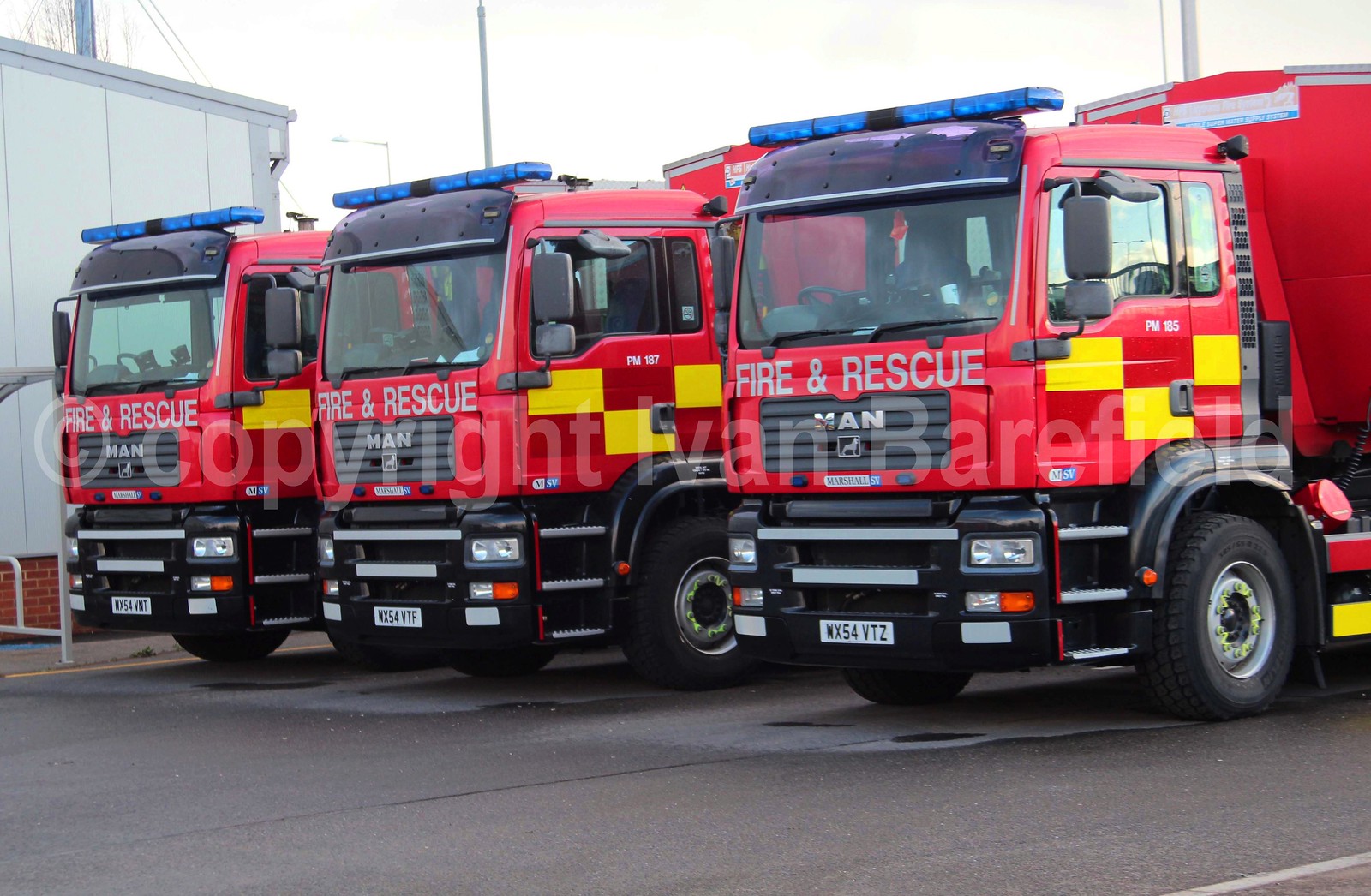This photograph captures three distinctive, bright red fire trucks lined up at an angle in a parking lot on a cloudy, possibly overcast day. Each truck prominently displays "Fire and Rescue" in gray lettering on the front. They feature red cabs and backs, black and silver bumpers, yellow and red checkerboard patterns on the doors, and blue lights on top. The trucks cut off just beyond the cabs, and are parked as if positioned for inspection or a demonstration, with the parking lot's gray asphalt wet, except under the vehicles. They appear non-American, likely German, as suggested by their unusual structure and Germanic license plates. To the left, the edge of a white building with a brick base is visible, and opposite, a red structure frames the scene. The atmosphere indicates recent or impending rain, adding a unique touch to the otherwise routine setting.